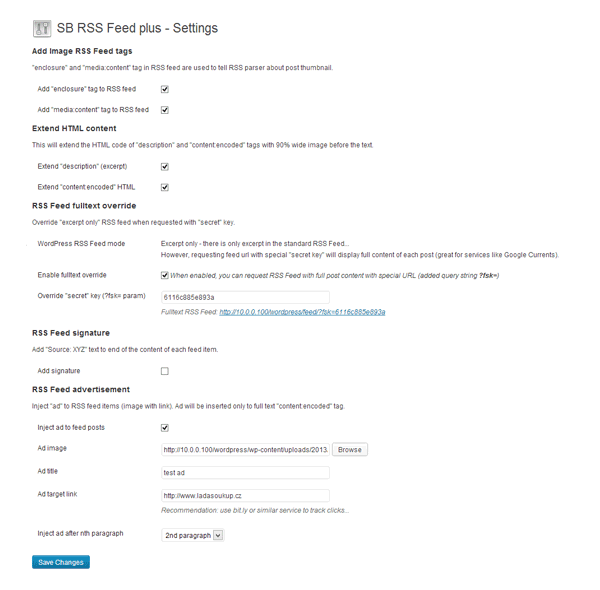The image depicts a computer screen displaying a settings page for "SB RSS Feed Plus." At the top of the page, the title reads "RSS Feed Plus - Settings." As you progress down the page, there are various options and settings related to RSS feed configuration.

First, there's a section labeled "Add image RSS feed tags," which includes an explanation: "Enclosure and media content tags in RSS feed are used to tell RSS parser about post thumbnail." Below this explanation, there are two checkboxes: "Add enclosure tag to RSS feed" and "Add media content tag to RSS feed," both of which are checked.

Further down, you notice that certain areas are highlighted in bold while others are in gray, indicating their status or importance. Towards the middle of the page, there is a clickable link formatted as "http://," suggesting it can be used for additional configurations or resources.

Continuing down, there's another section titled "RSS Feed Signature." Within this section, there's an option labeled "Add signature," which remains unchecked, while another option, "Inject add to feed post," is checked.

At the bottom of the settings page, there is a prominent blue button labeled "Save Changes," allowing the user to save their adjustments to the RSS feed settings. The overall appearance is designed to help users easily configure their RSS feed preferences.